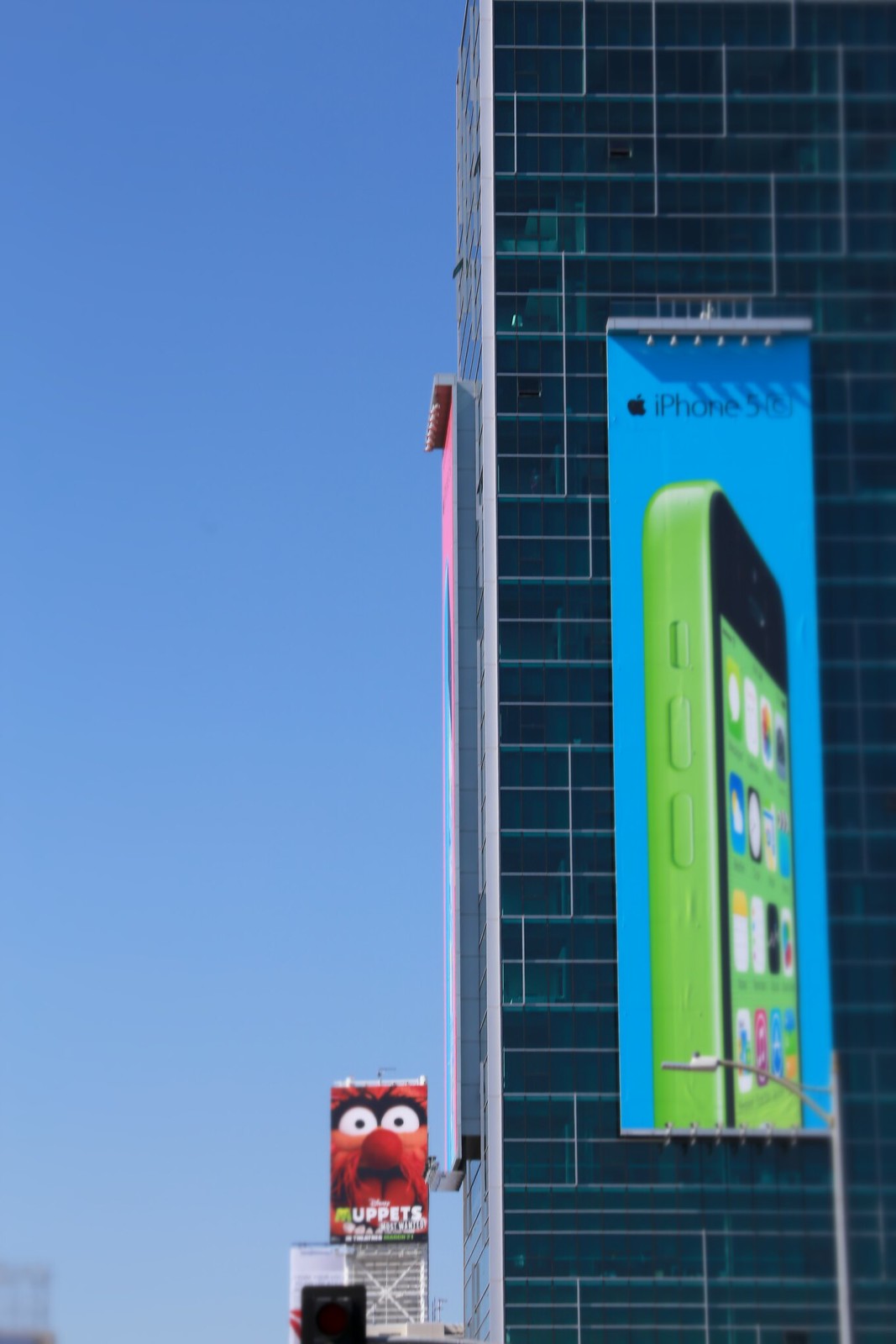A vibrant urban scene captured under a clear blue sky features multiple buildings adorned with striking advertisements. Dominating the right side of the image is a partially cut-off skyscraper, prominently displaying an iPhone 5C advertisement. This light green ad showcases the side profile of the phone angled to the right. To the left, though not fully visible, is another advertisement with a red background that is attached to the side of a neighboring building. In the distant background, towards the left but centrally located, stands another building with a white facade. This building, further away from the viewer, also sports an ad, this one promoting a Muppets movie. The combination of modern architecture and colorful advertisements creates a dynamic and bustling cityscape.